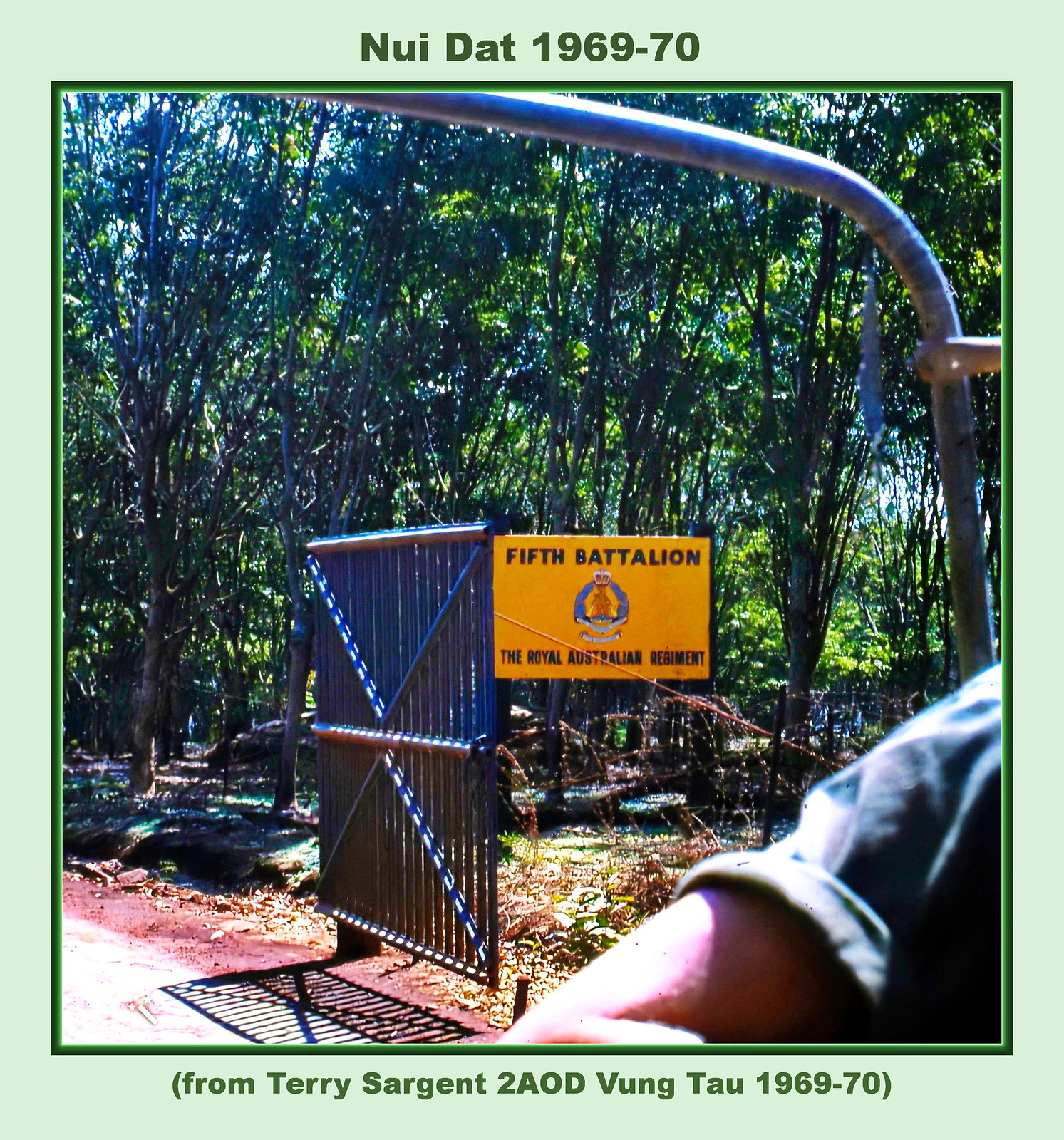The photograph, evidently taken during the Vietnam War, depicts an outdoor scene surrounded by a dense cluster of tropical, jungle-like trees. The foreground features a blue gate with a gold-colored sign, bearing the black or dark blue inscription "5th Battalion, the Royal Australian Regiment," along with a distinct symbol or logo. The setting includes a mixture of red dirt and pavement leading into the tree area, with a small area of water visible amid the vegetation. A curved pole, likely part of a vehicle, extends into the frame, and a person's arm is visible near the bottom edge. The image is bordered by a light green outer frame and a darker green inner frame. Text at the top and bottom reads "Nui Dat 1969-70" and "From Terry Sergeant to AOD, Vung Tau 1969-70" respectively, all in dark green or nearly black lettering. The sky peeks through the trees in the distant background, enhancing the natural, lush atmosphere of the scene.